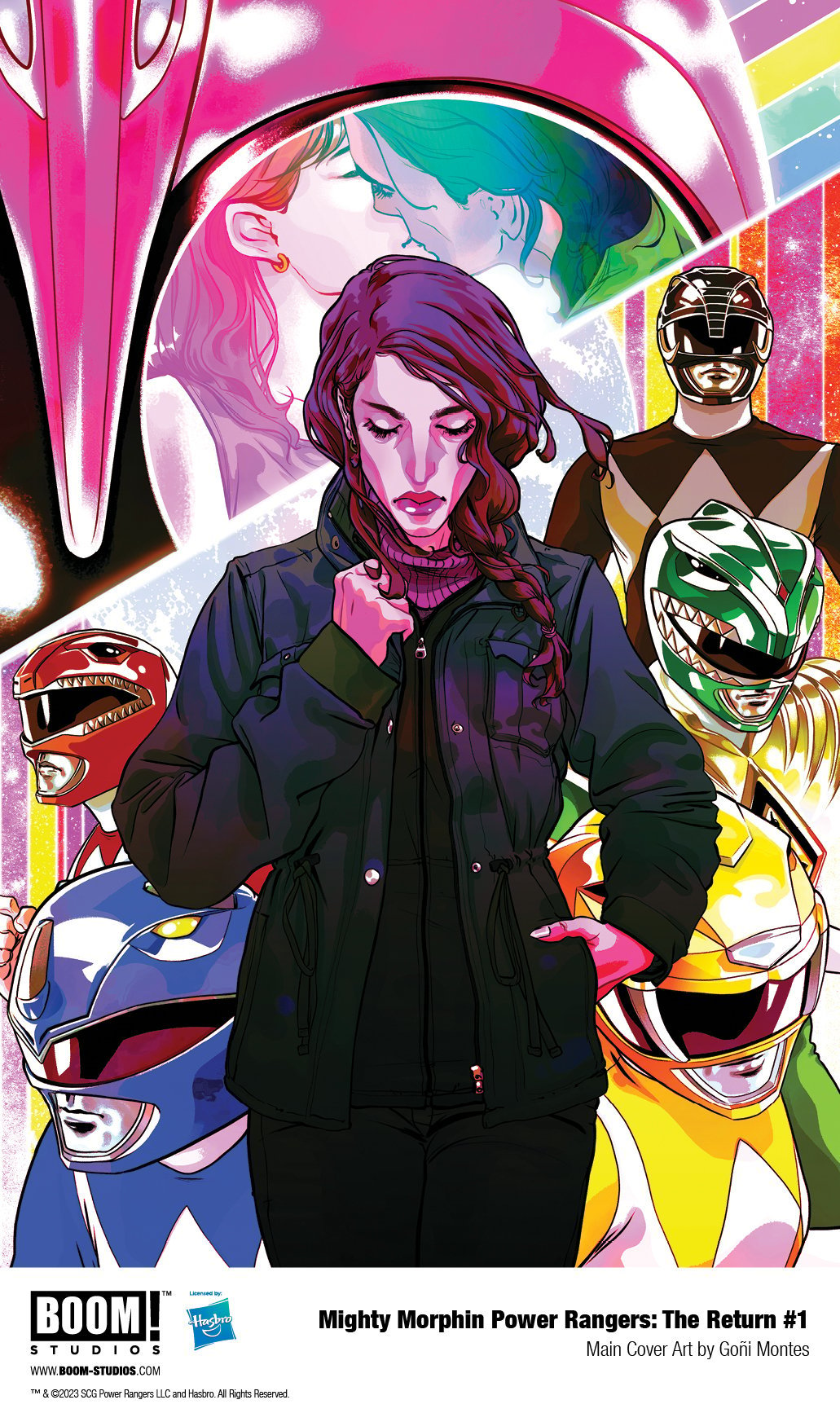This digitally-created poster, likely for a comic book or graphic novel cover titled "Mighty Morphin Power Rangers: The Return #1," features intricate and vibrant art. At the centerpiece is a woman with long purplish hair, dressed in a blue jacket, black turtleneck, and black pants. She clutches the collar of her jacket with her right hand, while her left hand is tucked into her pocket, with her thumb visible. Above her is a semicircle encapsulating an image of her kissing a man. The backdrop displays pink hues at the top with diagonal stripes in purple, yellow, and blue in the top right corner, adding a dynamic touch to the composition. 

Flanking the central figure are the Power Rangers: the blue and red Rangers are to her left, looking leftward, while the yellow, green, and black Rangers are positioned to her right, with the black Ranger looking straight ahead. At the bottom of the poster, "Boom Studios" and the Hasbro logo are present, alongside the text "Mighty Morphin Power Rangers: The Return #1" in black font, indicating this as an official product. Additionally, the cover art is credited to Goni Montas.